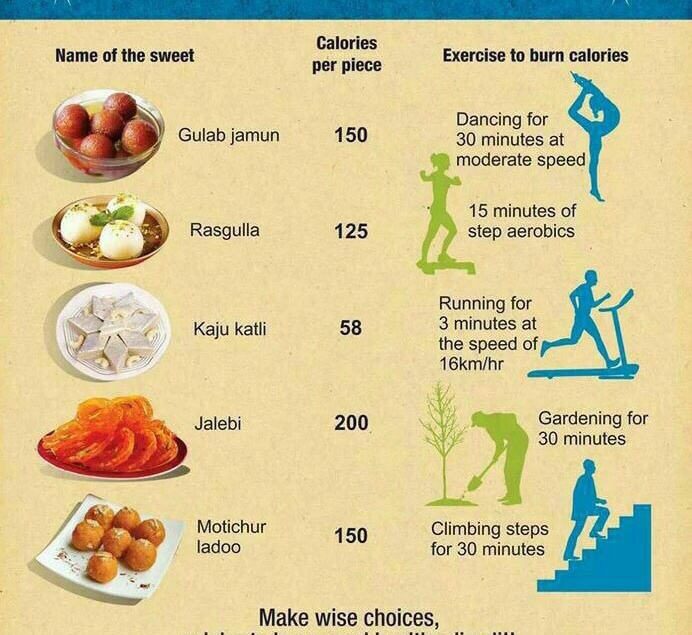The image is a detailed infographic with a tan background and a blue border at the top. It is divided into three rows: "Name of the Sweet," "Calories per Piece," and "Exercise to Burn Calories." Along the left side, there are pictures of various Indian sweets including Gulab Jamun, Rasgulla, Kaju Katli, Jalebi, and Motichur Laddu. Each sweet's calorie content and the corresponding exercise required to burn those calories are listed. 

Gulab Jamun contains 150 calories per piece, which can be burned off with 30 minutes of moderate-speed dancing. Rasgulla has 125 calories per piece, requiring 15 minutes of step aerobics to burn off. Kaju Katli, a white star-shaped sweet, contains 58 calories per piece, needing 3 minutes of running at 16 kilometers per hour. Jalebi, with 200 calories per piece, equates to 30 minutes of gardening to burn off, and Motichur Laddu, at 150 calories per piece, requires 30 minutes of climbing steps. 

There are small images illustrating these exercises: a girl dancing, a person on a treadmill, and someone gardening, depicted in blue and green. At the bottom of the chart, it advises readers to "Make Wise Choices," emphasizing the importance of healthy decision-making regarding sweet consumption and exercise.